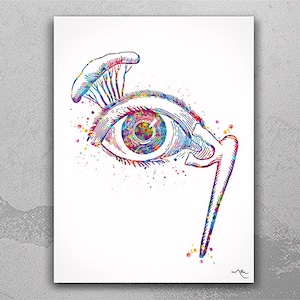This image features an abstract painting on a white canvas set against a light gray background that darkens towards the bottom, giving the impression of an elevated display. The canvas displays a striking eye motif, rendered in a rainbow of sparkly colors, which intriguingly merges with black and white tones. The central image comprises an eye with intricate detailing, including an iris, a surrounding circle, and a white outer section. Above the eye is an eyebrow with a predominantly white top.

On the left side of the canvas, branches extend upward from the top of the eyelid, capped with a cloud-like formation. On the right side, a mysterious object resembling a walking cane or pole with a claw-like end is attached to the eye. Surrounding the eye are dots and lines in purple, blue, and green, adding to the artwork's vibrant and otherworldly feel. The piece is signed in black freehand at the bottom right, though the signature is too small to be legible. The background's textured gray hues create an illusion of depth, enhancing the surreal and compelling nature of the artwork.